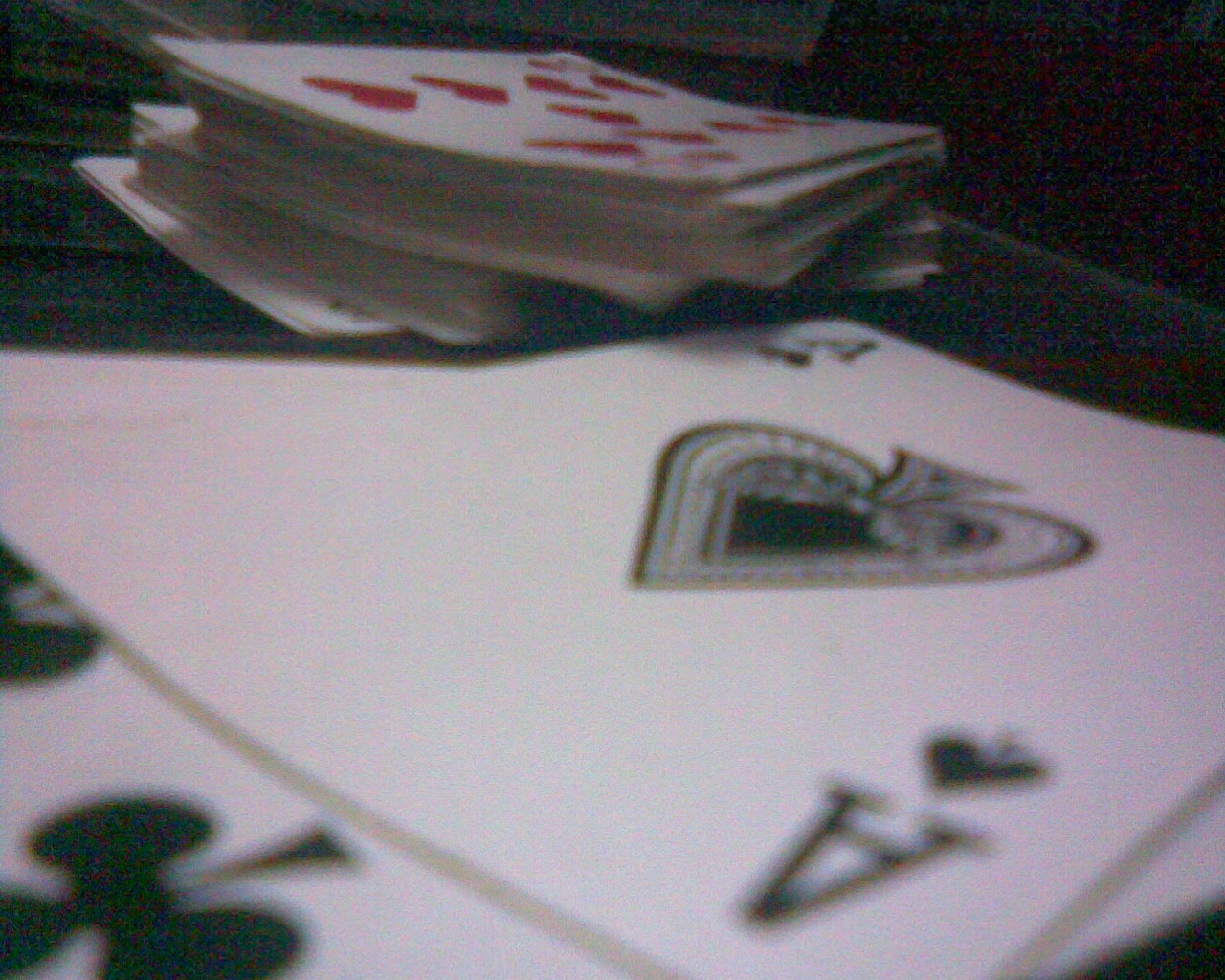In this close-up image of playing cards on a tabletop, the ace of spades takes center stage. The card's design is classic, with a prominent 'A' and a spade symbol at both the top and bottom corners. The centerpiece spade is intricately decorated, featuring a bold black outline with a dotted pattern inside. Partially hidden beneath the ace of spades, a clubs card peeks out, though its rank is not discernible. The surface under the cards is a black or dark gray color, marred by red and green visual artifacts that add a speckled distortion to the image. In the background, a haphazard stack of playing cards leans to one side, with a nine of hearts visible on top, identifiable by its nine heart symbols.